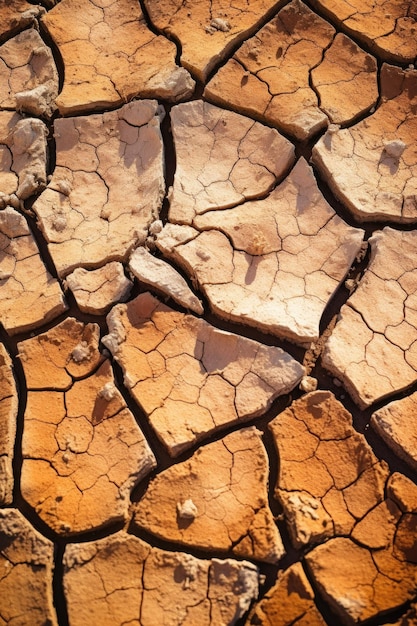The image portrays a close-up view of a parched, cracked expanse of soil, evocative of a dried-up lake bed or a desert landscape. The ground features extensive, winding cracks that crisscross and segment the surface into irregular, crisp-edged chunks. Predominantly brown, beige, and tan hues permeate the scene, accentuated by variations, including subtle yellows and occasional dark brown areas, lending depth to the parched earth. Small white pebbles are scattered across the terrain, introducing slight contrast to the predominantly warm color palette. Sunlight highlights certain sections, emphasizing the texture and relief of the dried, fragmented soil. The impression of a lifeless, moisture-deprived land is palpable, with the varying shades and intricate network of fissures enriching the intricate desolation depicted in the frame.